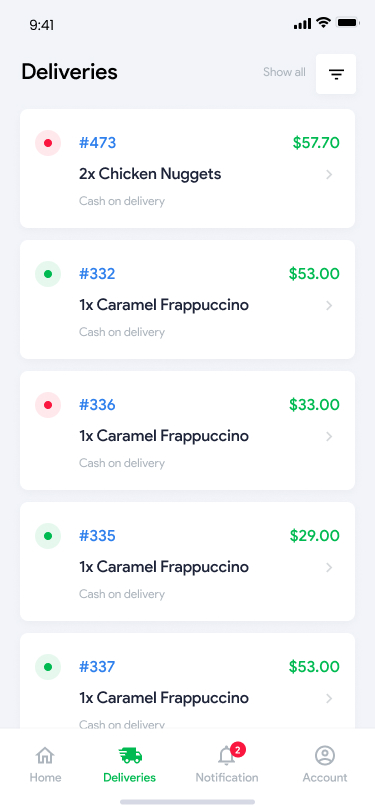This screenshot taken from a smartphone displays a delivery app interface. The time is shown as 9:41 AM in the upper left-hand corner on a white background. The status icons indicate full cellular signal bars, active Wi-Fi, and a fully charged battery. 

The screen primarily features a section labeled "Deliveries" in bold black text. Below this heading, the delivery details are listed:

1. Delivery #473: Two orders of chicken nuggets priced at $57 each.
2. Delivery #332: One caramel frappuccino priced at $53.
3. One caramel frappuccino priced at $33 with a notation of "cash on delivery."
4. Delivery #335: One caramel frappuccino priced at $29 with "cash on delivery."
5. Delivery #337: One caramel frappuccino priced at $53 with "cash on delivery."

Each delivery item is listed with its respective number and pricing details. Out of the five listed deliveries, three prices are highlighted in green, while two are marked in red, possibly indicating completed and pending deliveries, respectively.

Additionally, a green button labeled "Deliveries" is visible, indicating the user's current screen, alongside a notification icon with two unread messages. Below this, an "Account" option is available for user access.

This organized screenshot suggests the user is managing their delivery orders, tracking both successful and outstanding payments.